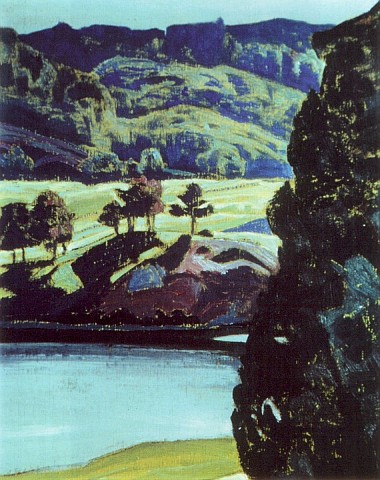The image depicts a surreal, painterly landscape with a turquoise blue body of water occupying the bottom left corner. The foreground features a bright green strip of grass, accompanied by a dark evergreen tree positioned prominently in the bottom right corner. A brownish boulder stands behind the turquoise water, casting shadows on a green hill dotted with small trees. Beyond this, the landscape transitions into rolling fields of grass interspersed with additional trees and hills, eventually giving way to blue and light green mountains. A sliver of sky is visible at the very top. The large, dark structure on the right, which could be either a tree or a rock formation, adds a sense of mystery to the composition. The scene evokes a dreamlike quality, almost reminiscent of a surreal golf course or a fantastical field with varied elevation and vivid colors.